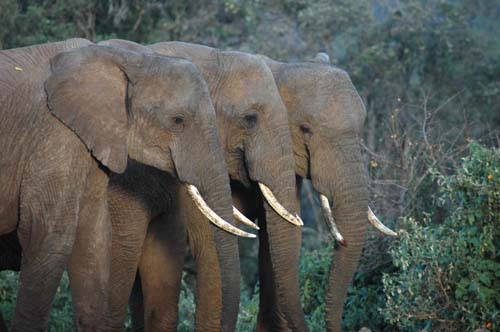The image depicts three large elephants standing side by side, taking up a significant portion of the frame. The photograph captures them from the side, showing their massive trunks, tusks, and the upper parts of their bodies. The first elephant, situated on the left side, displays tall legs, a long trunk, and white, though somewhat grayish, tusks extending from beneath its large ear. The second elephant stands directly behind the first, its legs hidden from view but with visible white tusks and a lengthy trunk. The third elephant, positioned behind the second, has its head slightly turned, revealing only one eye, along with its tusks and trunk. The elephants are set against a vibrant natural backdrop featuring trees with green leaves, bushes, brown branches, and scattered leaves both in the air and on the ground.